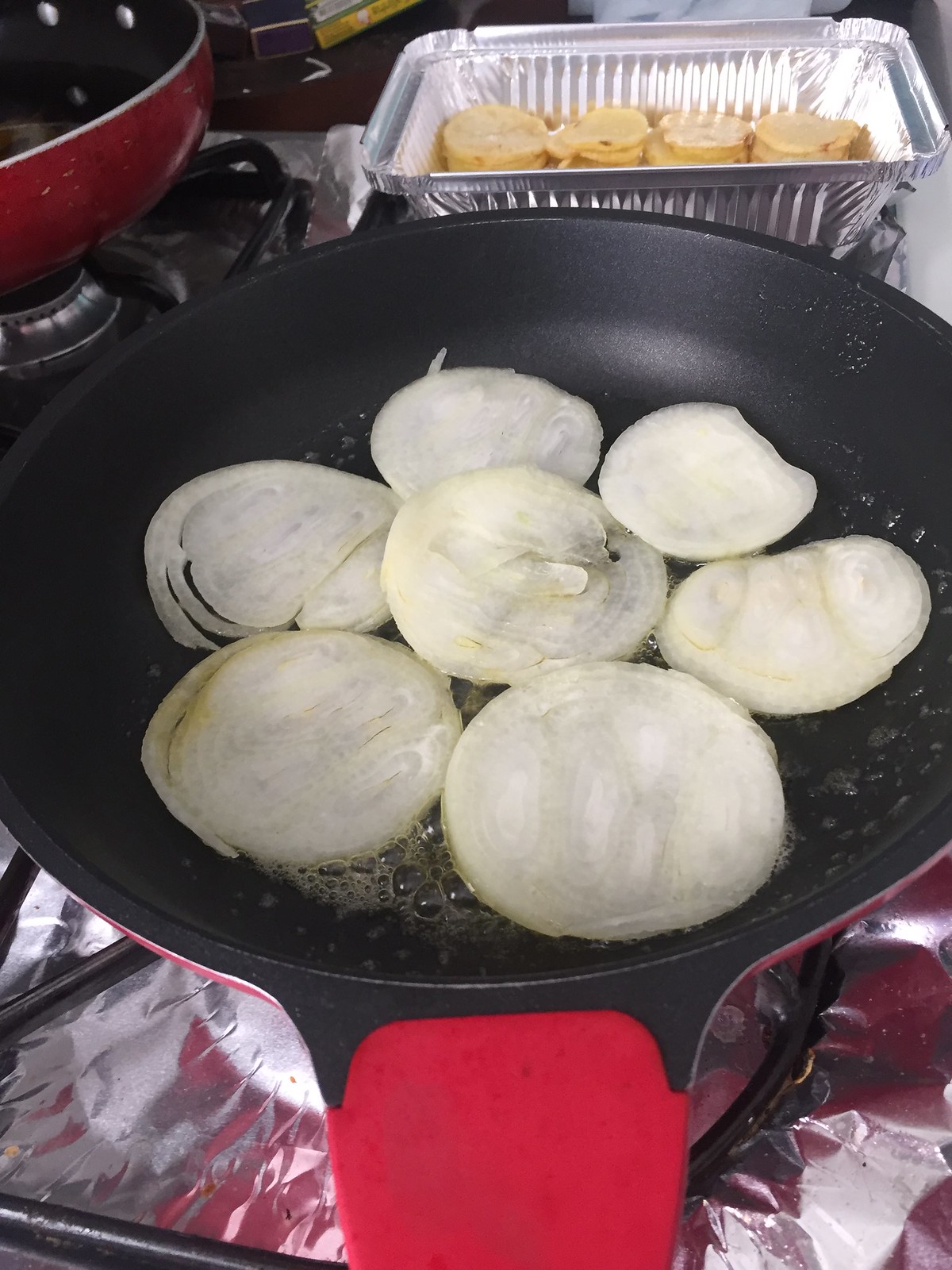The photograph captures a close-up scene of a kitchen stovetop. Central to the image is a red-handled frying pan with black sides, containing seven white onion slices arranged like a flower—one slice in the center surrounded by six in a circle. Melted butter at the bottom of the skillet is partially bubbling, creating foamy bubbles visible at the side closest to the viewer. The stove's burner is lined with bright silver aluminum foil, and additional foil covers the entire stovetop area. Behind the frying pan, there's a disposable aluminum container with yellow circular items, likely cooked onion slices. In the upper left corner of the photo, part of another red cookware piece, possibly a bowl or pan, is visible on a different burner.